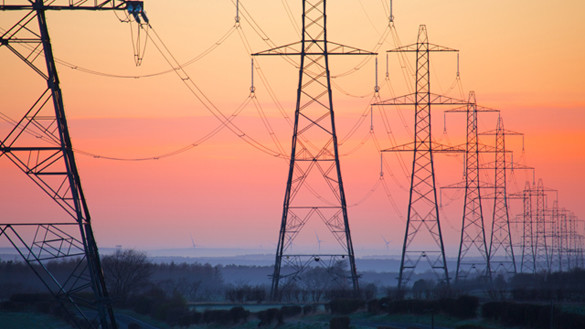This color photograph, horizontally oriented, captures a striking sunset skyline adorned with a series of tall metal pylons, possibly electric towers, stretching from the upper left to the lower right of the image. The towers are interconnected by sagging power lines that create a series of gently looping arcs. As the perspective draws the viewer's eye from the foreground to the background, the pylons diminish in perceived size due to the depth of field, contributing to an impression of endless continuity.

The sky is an enchanting gradient of sunset hues, transitioning from a pale orange at the top, blending into soft pinks, then to a more intense fluorescent orange and light yellows. Near the horizon, the colors deepen into a rich blue that outlines the shadowy silhouette of a distant cityscape and potentially some woodland or shrubbery. The bottom portion of the image retains the dark, in-shadow lines of the skyline, offering a stark, yet complementary contrast against the vibrant sky above.

In the far background, the faint shapes of buildings and possibly a port with cranes can be discerned, suggesting the setting is near a coastal city. The photograph exquisitely captures the grandeur and immensity of the pylons standing tall against a beautifully colored sky, with the loom of power lines symbolizing the connection and continuity that these structures bring to the urban landscape. The scene, devoid of any text or additional elements, purely focuses on the visual interplay of industrial utility and natural beauty at sunset.